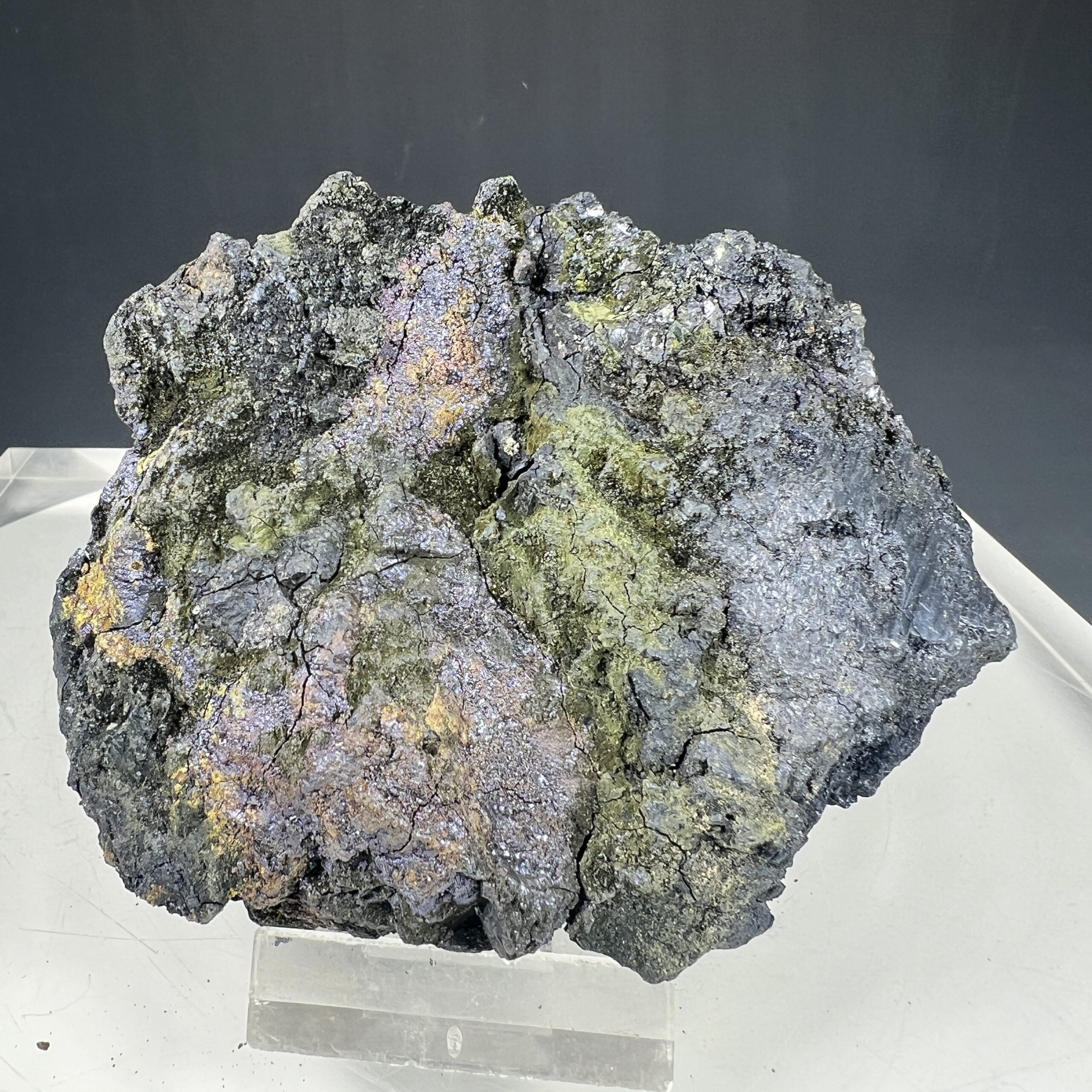This close-up photograph showcases a large, irregularly shaped rock or mineral with a highly textured surface. The rock features prominent cracks and a diverse color palette that includes grays, blacks, and blues, with noticeable splashes of green, and flecks of orange, gold, purple, and silver adding to its striking appearance. The rock's rough, cracked exterior suggests different sections that transition in color, emphasizing its complex structure. It is elevated on a clear glass stand above an unremarkable white table, appearing to dominate about 80-90% of the frame. The background of the image is predominantly black, providing a stark contrast that highlights the rock's intricate details and rich coloration.